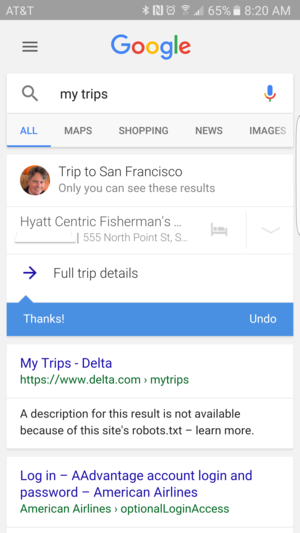The image depicts a smartphone screen at 8:20 AM with the battery level at 65%, utilizing AT&T as the service provider. The screen shows a Google search page with "Google" at the top, displayed in the brand's iconic colors (blue, red, yellow, and green). In the search bar, the user has typed "my trips."

Below the search bar, there are various category tabs labeled "All," "Maps," "Shopping," "News," and "Images." The "All" tab is highlighted in blue. The search results prominently feature a query for "trips to San Francisco," presenting detailed information regarding Hyacinth Rick Fisherman's located at 555 North Point Street.

A blue band labeled "Full trip details" appears beneath the address, accompanied by a "Thanks" button in white text and an "Undo" option on the right. The next result shows "My trips Delta" from Delta.com, although the description is not available because of the site's robots.txt settings. Below this, there's a prompt to log in to an AAdvantage account with fields for login and password, specifically for American Airlines.

The webpage features a mix of colors, including blue, red, yellow, green, black, gray, and white. The "My trips Delta" text is blue, while the website address appears in green. Descriptions are rendered in black, and the "Login AAdvantage account" and related text are in blue, with the login website address also in green.